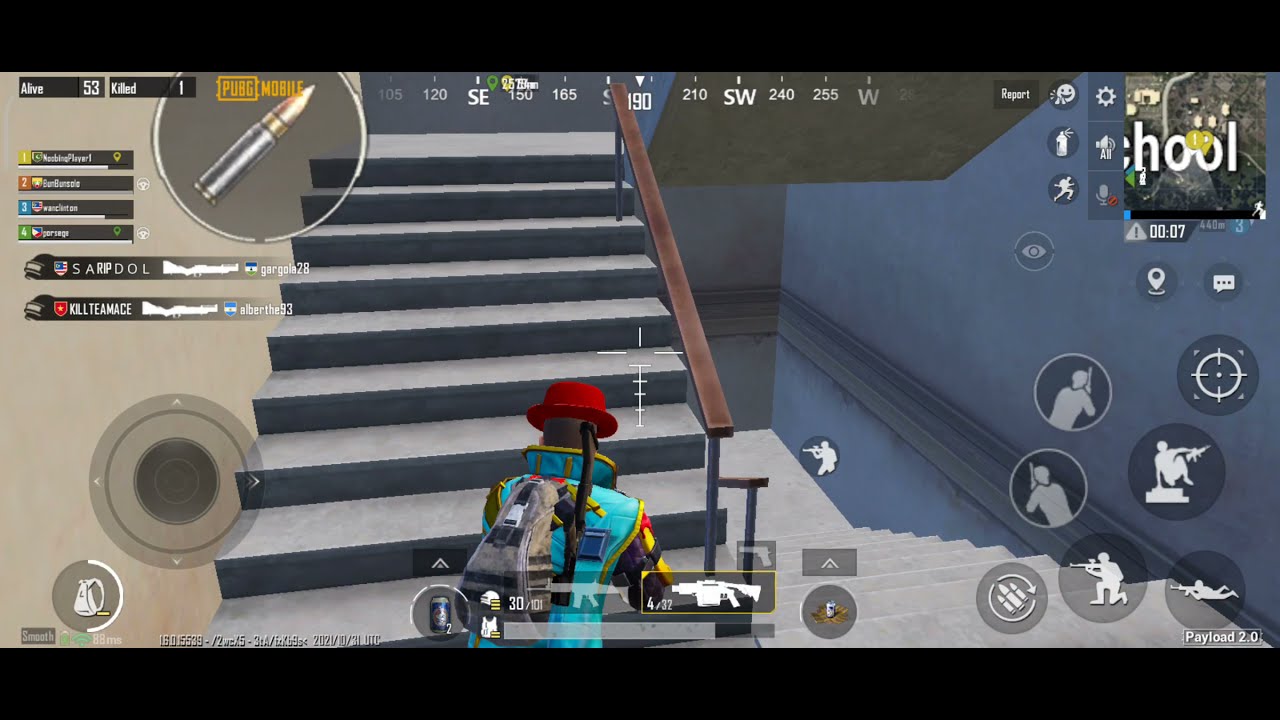The image depicts a scene from a third-person shooter video game, potentially Fortnite, characterized by its slightly cartoony aesthetic. The main character stands at the base of a gray staircase with a brown banister, ready to ascend. The character, wearing a distinctive red bowler hat, has long brown hair tied into a ponytail. They are clad in a light blue vest adorned with yellow trim around the collar and sleeves, along with a gray backpack fitted with tubes that run to the head. The overall environment is factory-like with bluish-gray tones dominating the scene. Various user interface elements are displayed: on the left side, icons indicate actions such as jumping, crouching, and shooting; on the right side, there's an icon showing the backpack's capacity and different available weapons. A compass is visible at the top of the screen, while a mini-map appears in the upper right-hand corner. The lower right-hand corner showcases different action options, reflecting a complex, interactive gameplay experience.